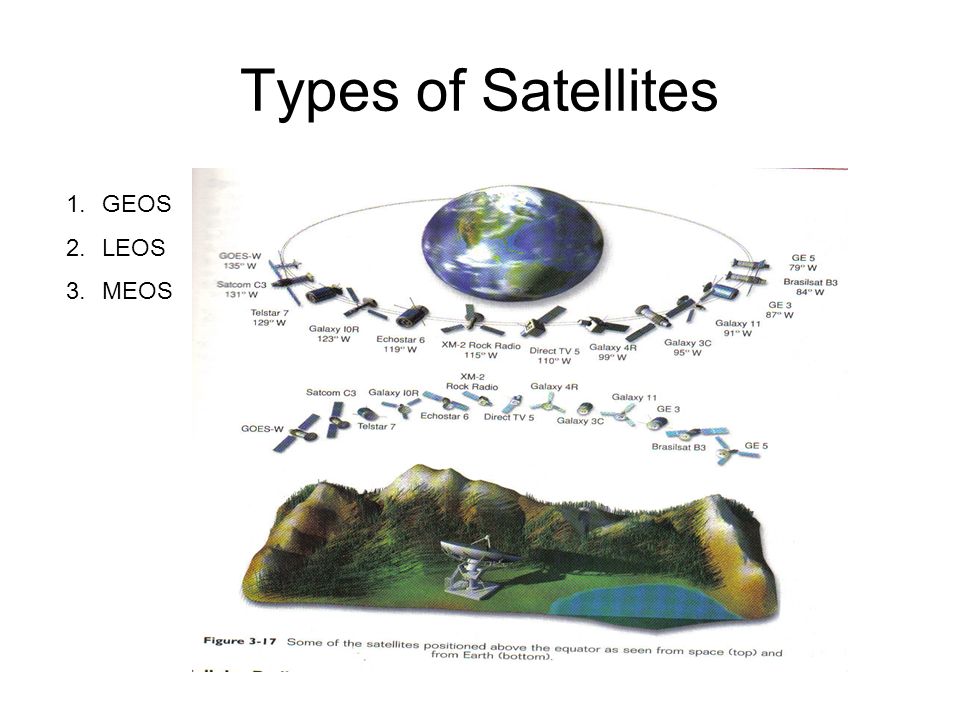The image is a detailed infographic titled "Types of Satellites" at the top. It features a central globe of the planet Earth, encircled by numerous satellites, displaying their coordinates in an elliptical orbit. On the left side, vertically aligned, are three bullet points numbered one, two, and three, labeled respectively as GEOS, LEOS, and MEOS. Thirteen satellites are depicted orbiting around the globe, with precise coordinates like GEOS at 130 degrees west and Galaxy IOR at 123 degrees west, indicating their positions. Below this main diagram, additional satellites, possibly the same thirteen, are shown. At the very bottom, there's an image of Earth with a satellite dish positioned in a grassy, mountainous terrain near a small lake. The dish appears to be communicating with the satellites above. The caption underneath this bottom image reads, "Figure 317: some of the satellites positioned above the equator as seen from space (top) and from Earth (bottom)."